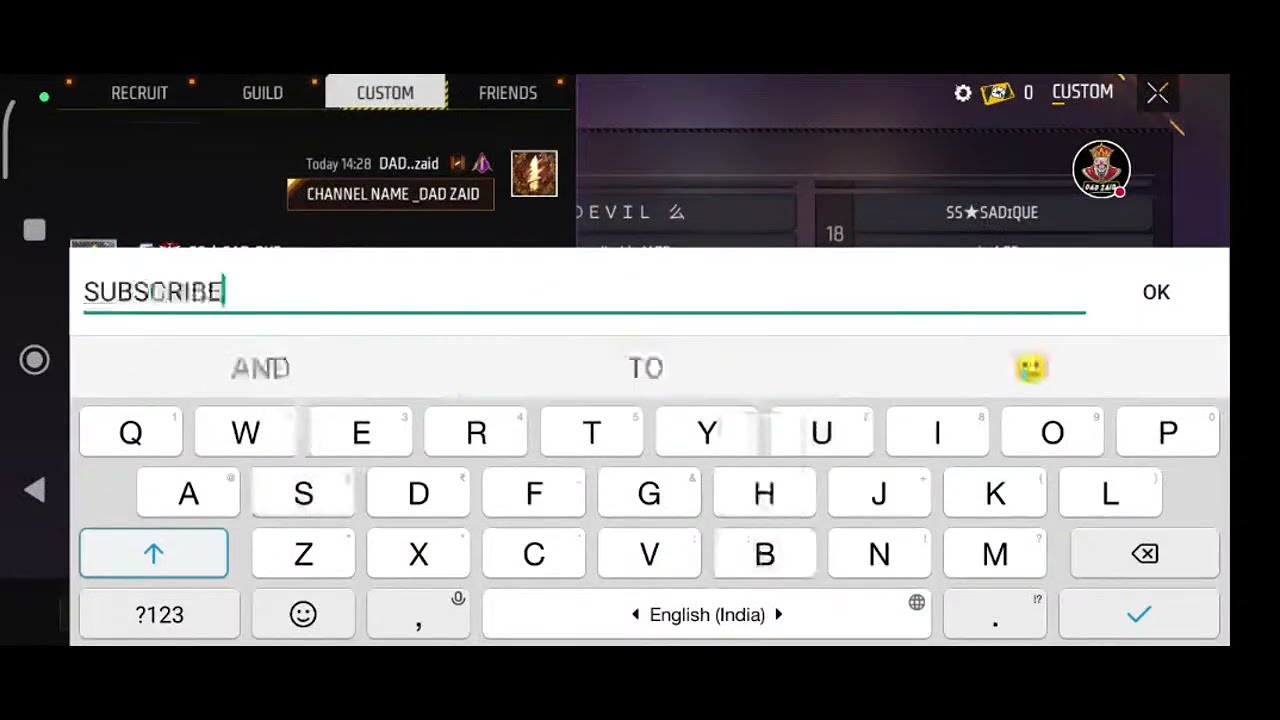The image is a horizontal screenshot displaying a virtual QWERTY keyboard on a mobile device, suggesting a dark-themed video game interface. The keyboard, occupying the bottom two-thirds of the image, features English letters in a light gray color. In the top left corner of the image, the text "SUBSCRIBE" is shown in black with a green underline and a green cursor positioned to its right. Above the keyboard area, there's a dark bar with white text that reads "RECRUIT, GUILD, CUSTOM, FRIENDS," with "CUSTOM" highlighted, indicating the current selection. Below this, it says "DADZRAID" and "CHANNEL NAME _ DADZADE." The top right corner features a circular cog, possibly a settings icon, and nearby icons for a masked character with a hat and the text "CUSTOM" accompanied by a number zero. Additional elements include a black square with a white 'X' to close the section and scattered geometric shapes like a square, circle, and triangle on the left side. The entire scene is set against a dark purple and black backdrop.